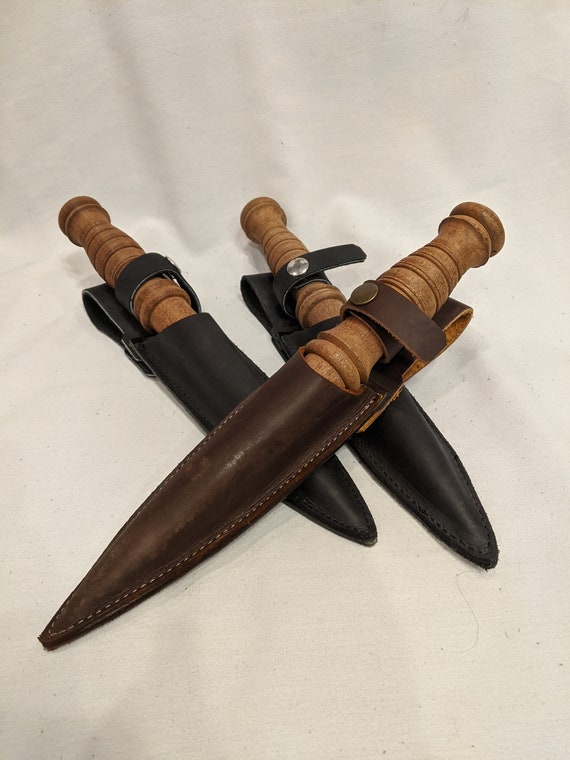The photograph showcases three intricately designed wooden practice daggers, each sheathed in leather. The daggers are arranged on a white cloth background, with two positioned horizontally at the bottom and one laid diagonally across the top. The horizontal daggers are housed in black or very dark brown leather sheaths, while the diagonal one is in a slightly lighter brown leather sheath. The sheaths feature closures, with a prominent white or silver snap on the rightmost bottom sheath and a tarnished gold snap on the top sheath, which also displays visible stitching around the edges. The handles of the daggers, likely round and lathe-turned, exhibit detailed carvings, adding to their elaborate appearance despite the low lighting and contrast.